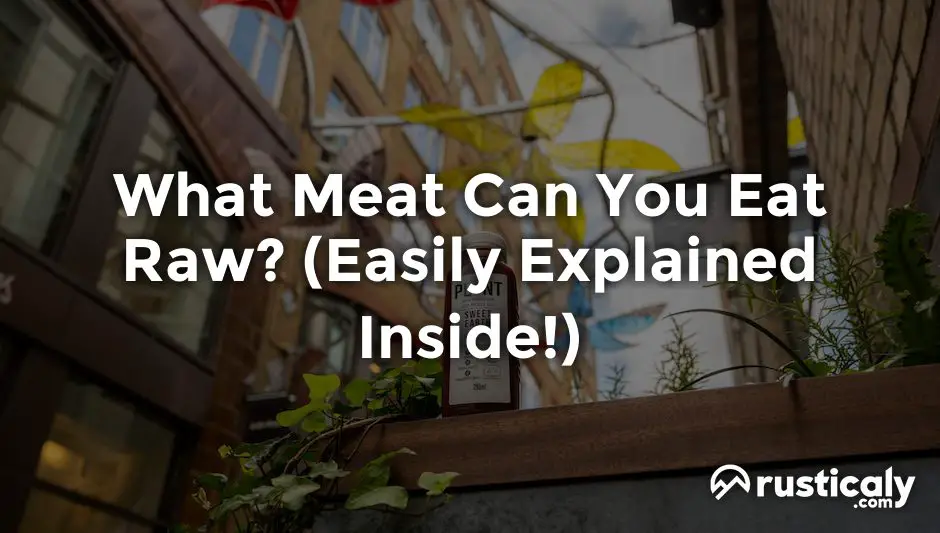The image is an advertisement for the website "Rusticly.com," showcasing the text "What meat can you eat raw (easily explained inside!)" prominently in white letters across the center. The background is a blurry, dark image featuring a brick building with windows on the left and a brick wall on the right, with green leaves and plants visible in the center. In the bottom right-hand corner, the website name "Rusticly.com" is displayed in white letters beside a circular logo that resembles a sun partially obscured by mountains. The scene appears to be an alleyway between two buildings, with additional details suggesting a blend of natural and urban elements, like a faint cloudy sky above. The entire image carries a rustic, serene aesthetic hinted at by the website's name and theme.